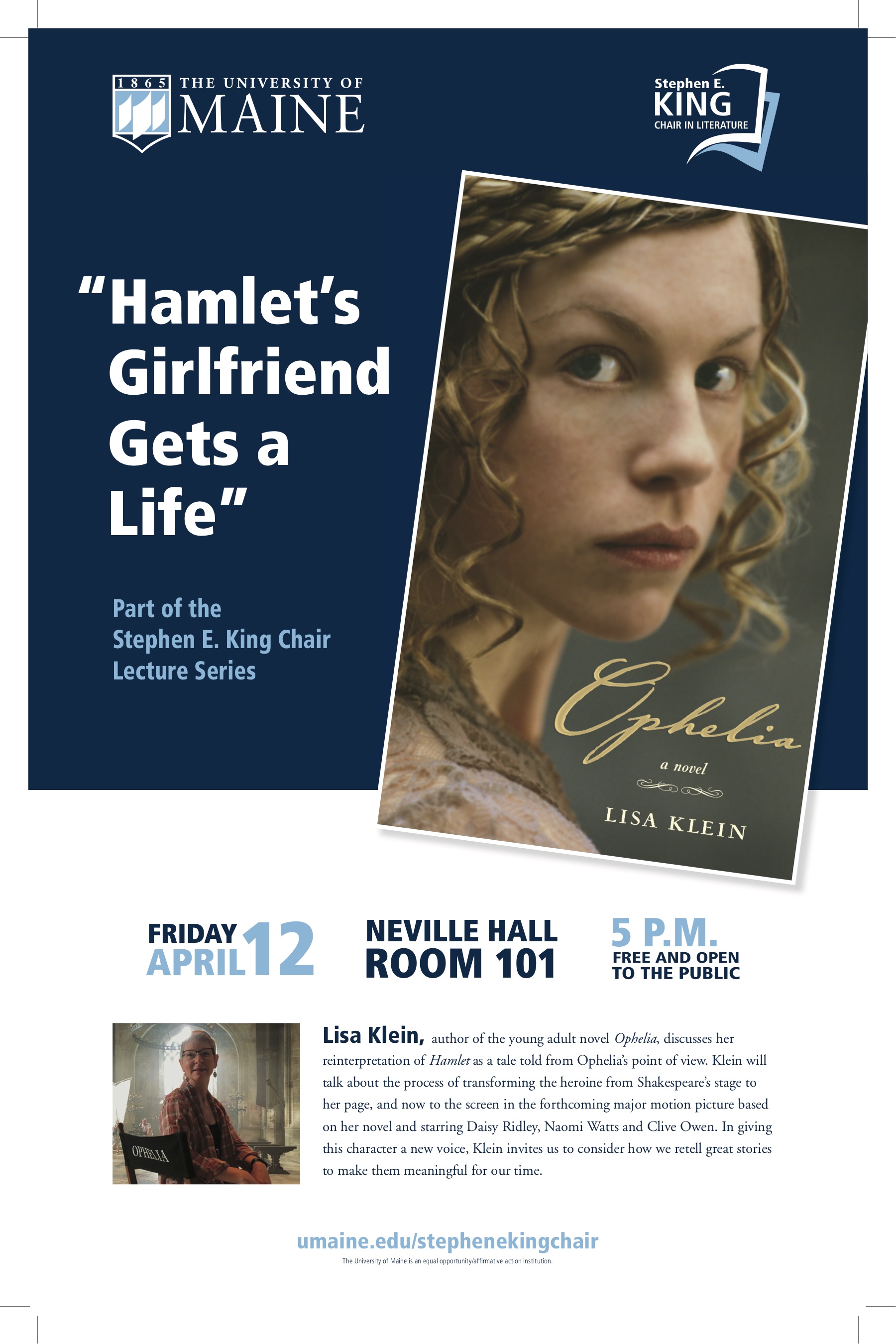The flyer from the University of Maine promotes an event titled "Hamlet's Girlfriend Gets a Life," as part of the Stephen E. King Chair Lecture Series. Featured on the flyer is an image of a young woman with blonde, spirally curls wearing a brown and beige floral dress, shown from the shoulders up. Additional imagery includes a small picture of author Lisa Klein, an older woman with white hair and glasses, sitting in a chair labeled "Ophelia."

The flyer details that on Friday, April 12th, at 5 p.m., in Neville Hall, Room 101, Lisa Klein will discuss her young adult novel "Ophelia," which reinterprets Shakespeare's "Hamlet" from Ophelia's point of view. Klein will elucidate the process of transforming this Shakespearean heroine from stage to page, and the creation of this novel, which can be seen as a form of fan fiction. This event is free and open to the public, and more information can be found at umaine.edu/stephenkingchair.